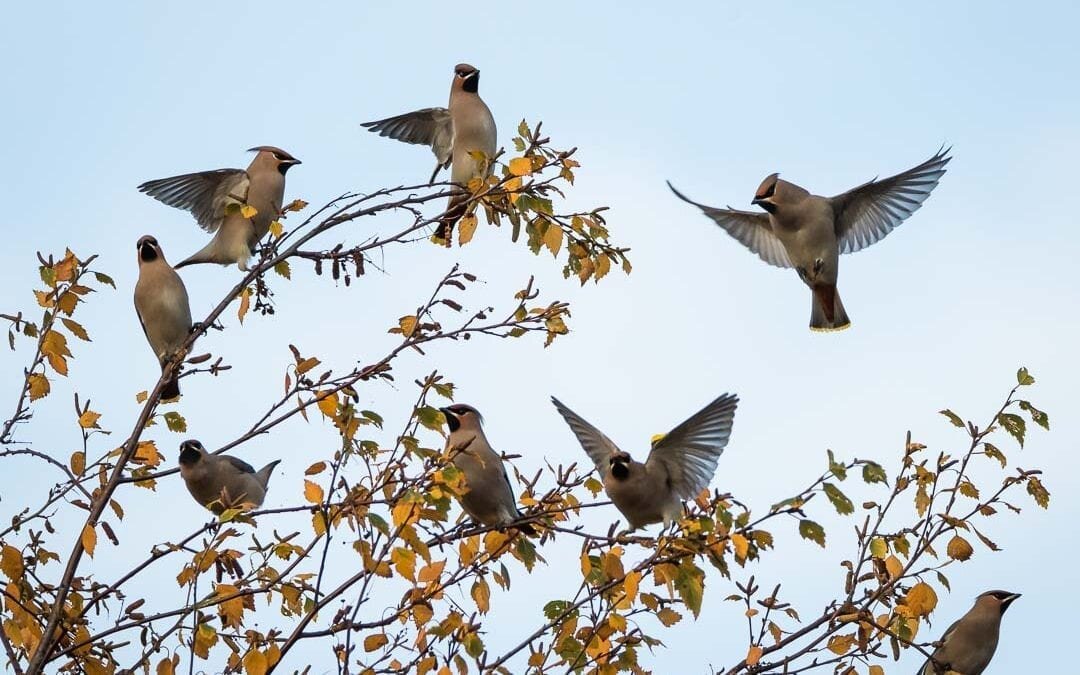A daytime photograph with a partly cloudy, light blue sky features a captivating sequence involving what appears to be the same blue and gray bird, possibly a Blue Jay, depicted in various stages of flight and rest. The image is meticulously edited to illustrate a dynamic time-lapse effect, showing the bird's graceful landing on, and subsequent departure from, a tree branch.

From right to left, the sequence begins with a bird mid-air, descending towards the branch. The next bird in the sequence is captured just as its wings are still arched upwards, finalizing its landing. Following this, another bird is perched serenely, gazing towards the left of the frame. Moving along, a bird is seen further on the branch, with three more birds positioned on a higher branch to the right, seemingly preparing for another takeoff, completing the sense of movement across the scene.

The composition of the image, juxtaposing the birds against the soft-colored sky, not only provides a stunning visual narrative of the bird’s motions but also highlights the natural beauty and elegance of avian life.